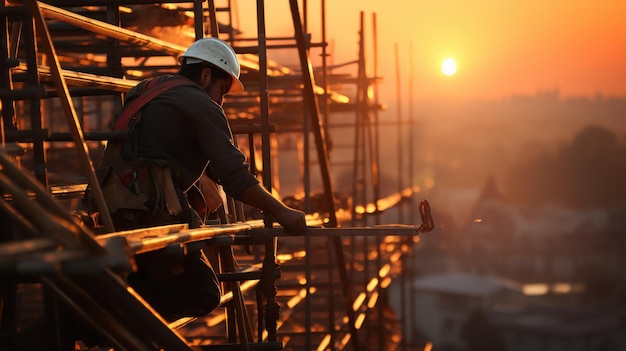The photograph captures a lone construction worker high up on the scaffolding against the brilliant backdrop of a sunset. He is dressed in a gray long-sleeve shirt with the sleeves pushed up, black pants, and a white hard hat. A safety harness with a red-orange strap runs down the middle of his back, and he has a tool belt around his waist. This worker is seen leaning over, focusing intently on a pole or a piece of the structure in front of him. His right hand grips the scaffolding's railing for support. The scaffolding itself is a complex network of tubing and walkways, with visible wood pieces and cross braces suggesting an ongoing build. In the background, the entire sky glows a vibrant orange, highlighting the silhouettes of distant buildings and trees, with the sun appearing as a small, bright circle just above the horizon. The scene beautifully juxtaposes the industrious activity with the serene, glowing light of the setting sun.